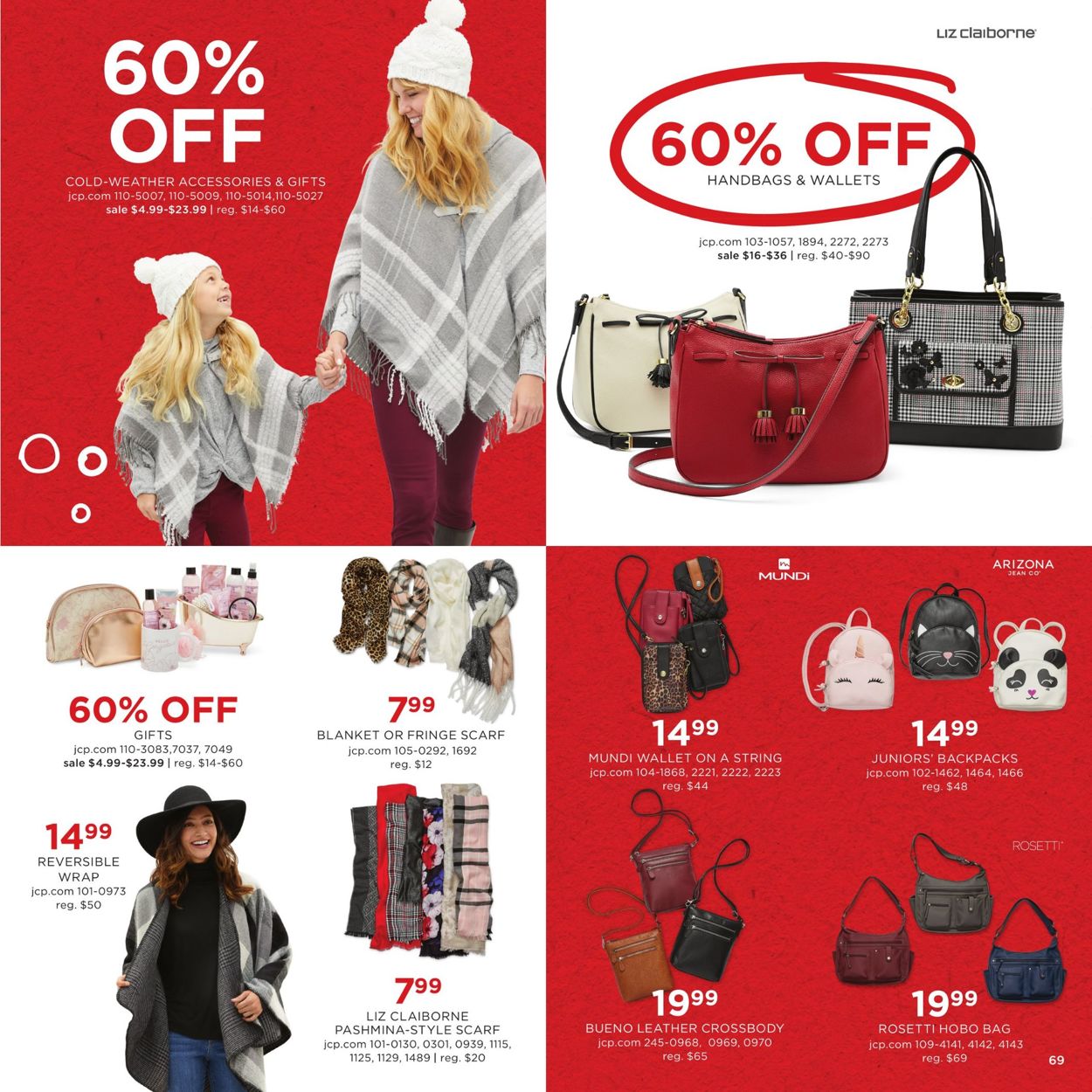The image is a vertical rectangular advertisement, slightly taller than it is wide, divided into four quadrants promoting a Christmas sale. The top left quadrant features a blonde woman and a blonde girl, both dressed identically in gray and white striped shawls, white stocking caps, and purple pants, looking at each other. The background is red with "60% off" displayed in white text.

In the top right quadrant, a red circle contains the text "60% off" in white. Below this, three purses are showcased: a white one on the left, a red one in the middle, and a gray and black one on the right, all set against a white background.

The bottom left quadrant displays a variety of items, segmented accordingly. The left section shows assorted purses and scarves, whereas the central focus is on clothing items, slightly obscured, with prices listed. The right section likely shows an assortment of scarves, initially mistaken for towels.

In the bottom right quadrant, an assortment of backpacks and various types of bags, including two distinct purses, are displayed. The background here is red, maintaining a cohesive festive theme throughout the advertisement.